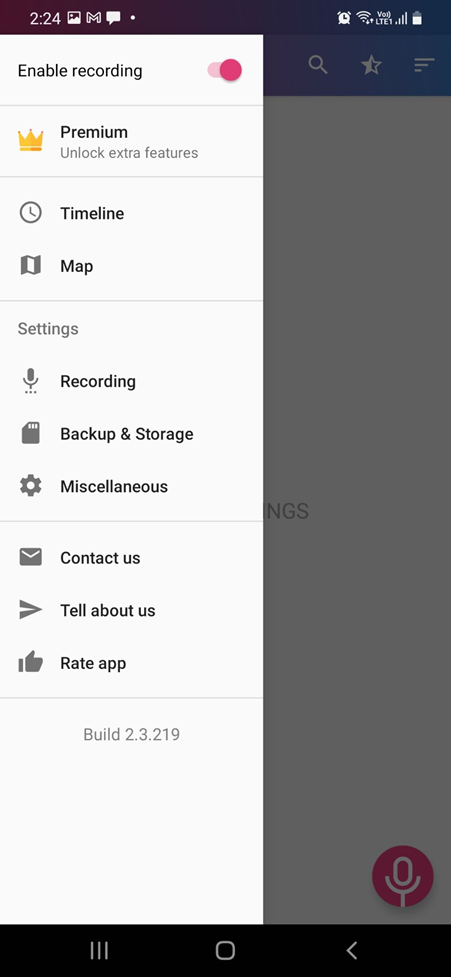The image displays a screenshot from an Android phone showcasing a music or audio recording application. At the top, a black status bar presents various notifications and system indicators. On the far left, the current time reads 2:24, and adjacent to it, there are icons for text messages, Gmail (an "M" icon), and other unread notifications. On the right side, icons display the phone's signal strength, data connection status, and battery level, which is approximately three-quarters full.

The main body of the image centers around the app's interface. Dominating the left side is a vertical white menu listing several options in black text, useful for navigating the app's features. The options, from top to bottom, include: "Enable Recording," "Premium," "Timeline," "Map," "Recording," "Backup and Storage," "Miscellaneous," "Contact Us," "Tell About Us," and "Rate App." At the menu's base, the text "Build 2.3.219" indicates the version number of the app. The "Enable Recording" option at the top features a pink box with a slider that is engaged, signifying that recording is active. 

On the bottom right, a conspicuous pink circle encloses a white stylized microphone icon, suggesting that tapping this will initiate a recording session. The app's suite of options evidently supports various functions such as recording, editing, storing audio files, and offering user support and feedback mechanisms. Despite the detailed interface, the app's name isn’t discernible from the screenshot.